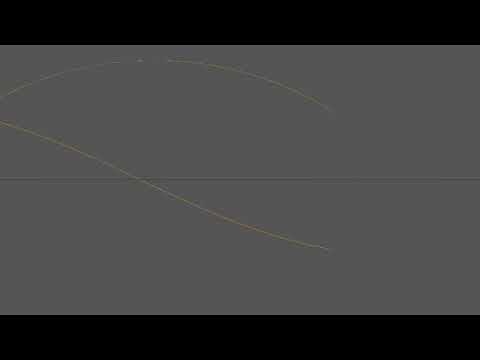The image is predominantly a dark gray rectangle framed by black bars at the top and bottom, each covering about a fifth of the total view. In the middle of this dark gray area, there is a noticeable horizontal seam or line that juts out like a folded piece of paper, extending halfway across the image. Towards the upper left quadrant of the gray area, there are two distinct markings. One of these markings arcs upward before curving back down, resembling the shape of an eyebrow and extending about three-fourths of the way to the right. The other marking descends diagonally to the bottom right, crossing over the horizontal seam and ending before reaching the bottom edge. These lines give the impression of scratch marks or contrails in the sky, adding an abstract texture to the otherwise monotone surface.